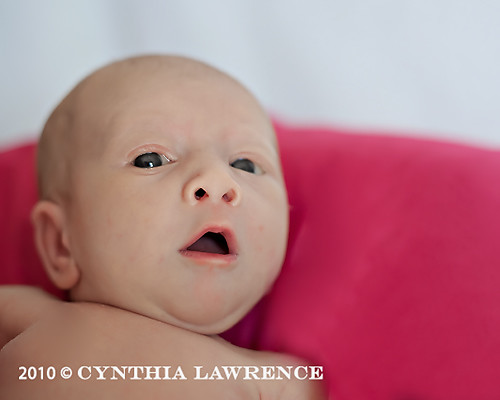The image showcases a newborn baby with dark eyes, very little hair, and a round face, lying on a pinkish-red pillow against a white background. The baby has an open mouth with pink lips, which accentuates a double chin, and a wide nose. Positioned prominently on the right side of the baby's head is a visible ear. The baby appears to be looking curiously up at the camera, giving an inquisitive expression. The baby’s chest is bare, and no hands or arms are shown in the picture. In the lower-left corner, there's white text that reads, "2010 © Cynthia Lawrence." The baby is placed mostly on the left side of the frame, with the white sheet or wall serving as the backdrop.